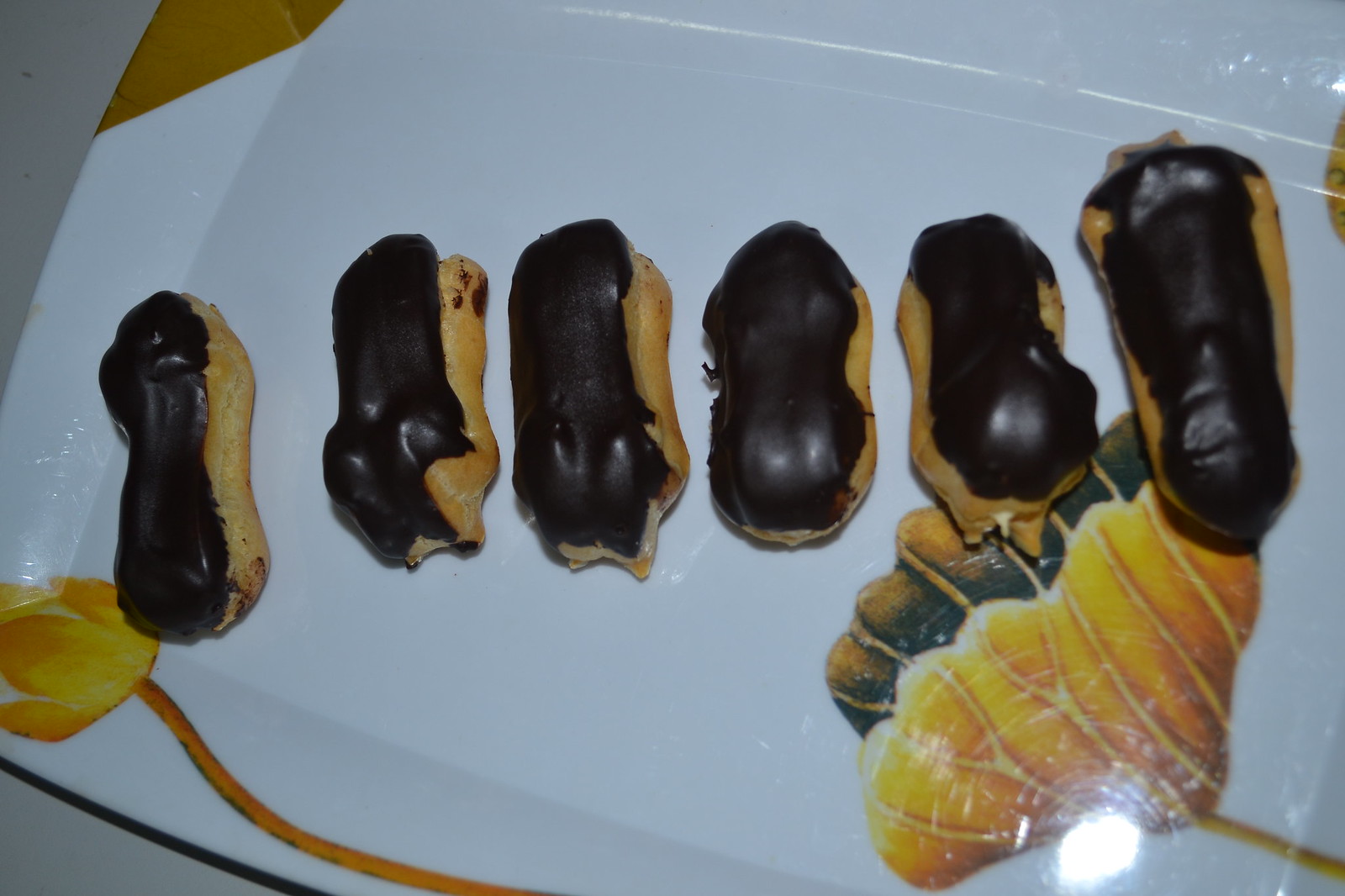The image shows a close-up of a beige- or gray-surfaced table, topped with a partially visible rectangular glass plate with an indentation in its center. This glass plate supports a white ceramic plate featuring a yellow and orange floral design, including an orange flower and a leaf with visible veins. The main focus is on six beige-colored, homemade eclairs with dark brown chocolate tops, aligned on the plate. The eclairs vary in size and shape, some appearing slightly peanut-shaped or oval, with one showing a bit of cream dripping from the bottom. The plate also displays additional orange and brown patterns around its edges, enhancing its decorative appearance.